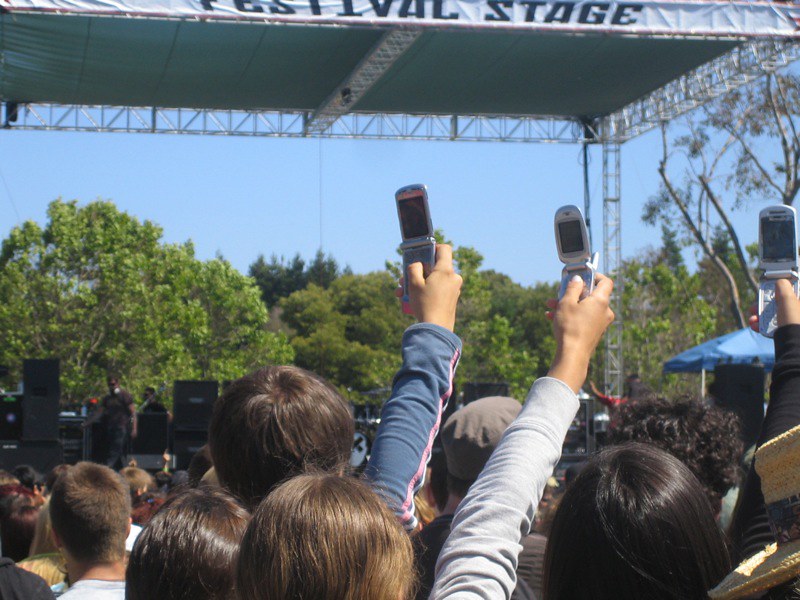This outdoor photograph captures a daytime musical concert from the back of a small crowd of spectators. In the foreground, three individuals are prominently holding up old-style flip phones, likely taking pictures or videos. The flip phones vary in design, with one appearing particularly stubby with an antenna, while the others are more flat or in between in shape. The arms holding these phones wear long sleeves, and the thumbs are positioned on the central controls of the devices.

The stage at the front of the crowd features large black speakers, musical amplifiers, and various equipment. Crew members are visible on stage, one walking to the left and another on the right. A white banner along the edge of the elevated metal structure covering the stage reads "festival stage." The cover is supported by exposed steel scaffolding and beams, with some cables hanging down and a blue shade umbrella placed towards the right middle of the image.

Beyond the stage, a dense backdrop of trees stretches towards the horizon under a clear blue sky, marking a picturesque natural setting that contrasts with the vibrant, technology-driven activities of the concert-goers.